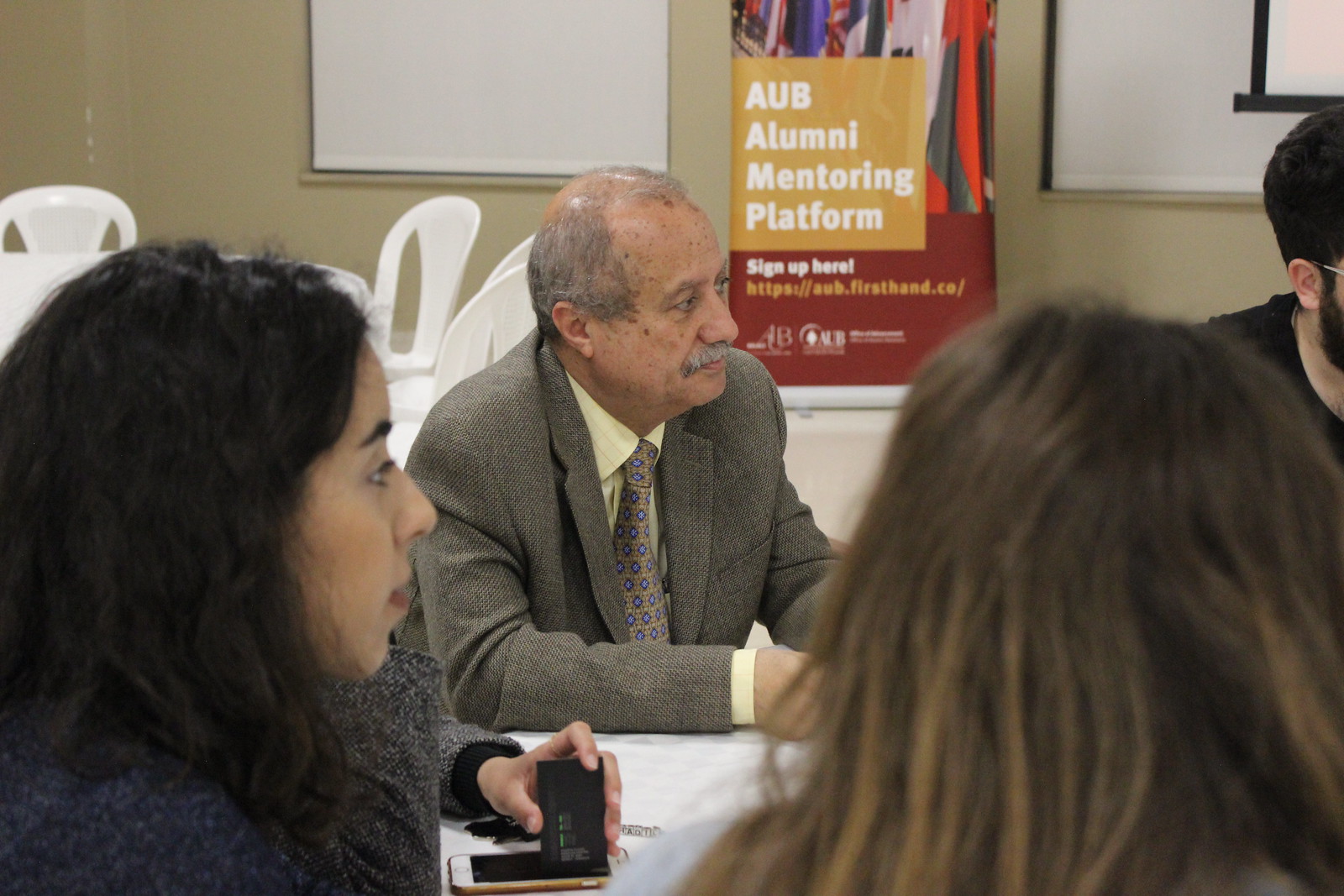The photograph captures an old man with a balding head, gray to white hair, and a gray mustache, sitting at a white table. He is dressed in a gray suit paired with a light-colored shirt and a tie featuring a spotted or star pattern. The scene is set within a room that resembles a meeting or classroom setting with some plastic chairs visible in the background. Directly behind the old man, there is a sign with golden yellow and maroon hues in parts, reading "AUB Alumni Mentoring Platform." In the foreground, two young women are partially in the frame: the one on the left has raven-black hair, and the one on the right is a light brunette. A hand, holding a black device that looks like a tape recorder, also appears on the table, partially obscuring the old man. The group seems focused on something to the right, outside the frame of the photograph.